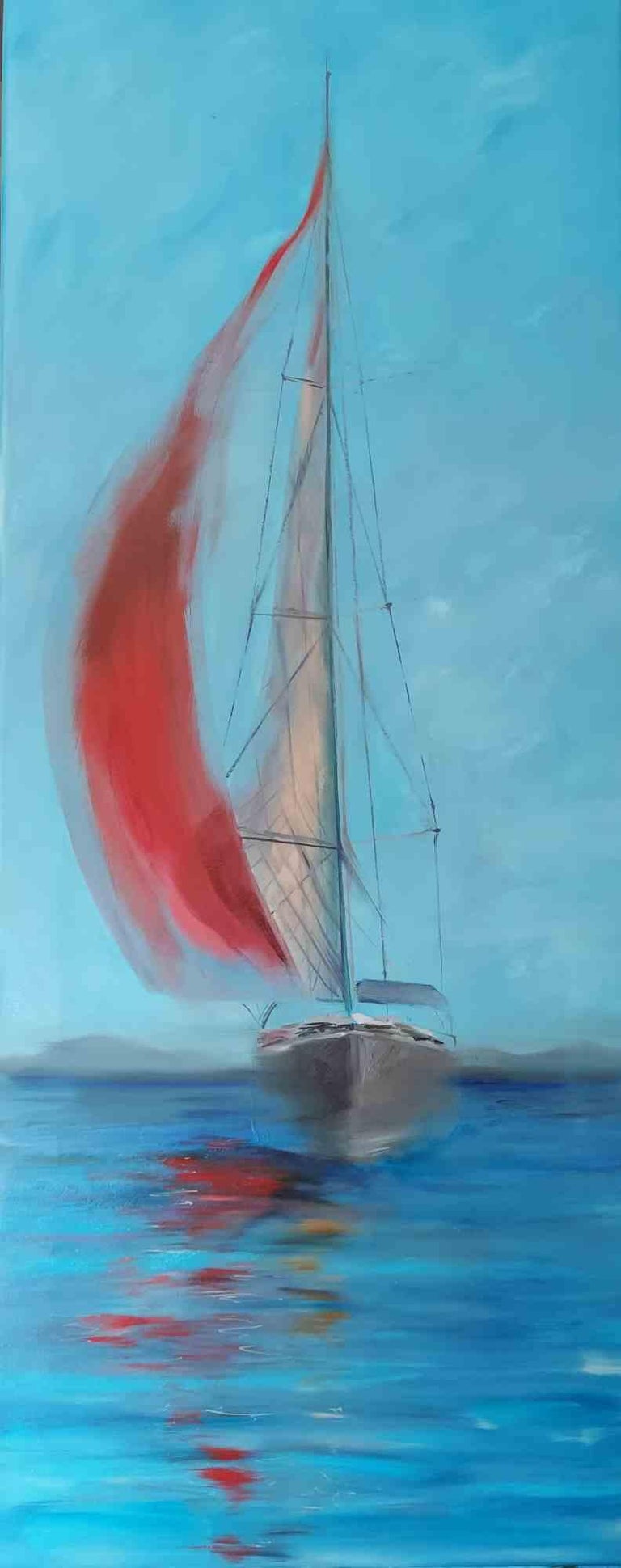In this painting, the viewer is captivated by the image of a sailboat navigating towards them. The visual centerpiece is undoubtedly the sailboat’s striking giant red sail, billowing robustly in the wind. Complementing it is a smaller, white sail that appears less taut, trailing behind. The ethereal ambiance of the scene is accentuated by the water, which merges almost seamlessly with the sky, evoking a surreal atmosphere. The water’s surface is particularly mesmerizing, reflecting both the vivid red sail and the sailboat with a shimmering clarity that blurs the boundary between water and sky. This play of light and color not only enhances the painting's dreamy quality but also underscores the artist’s intent to evoke a sense of peacefulness and wonder.